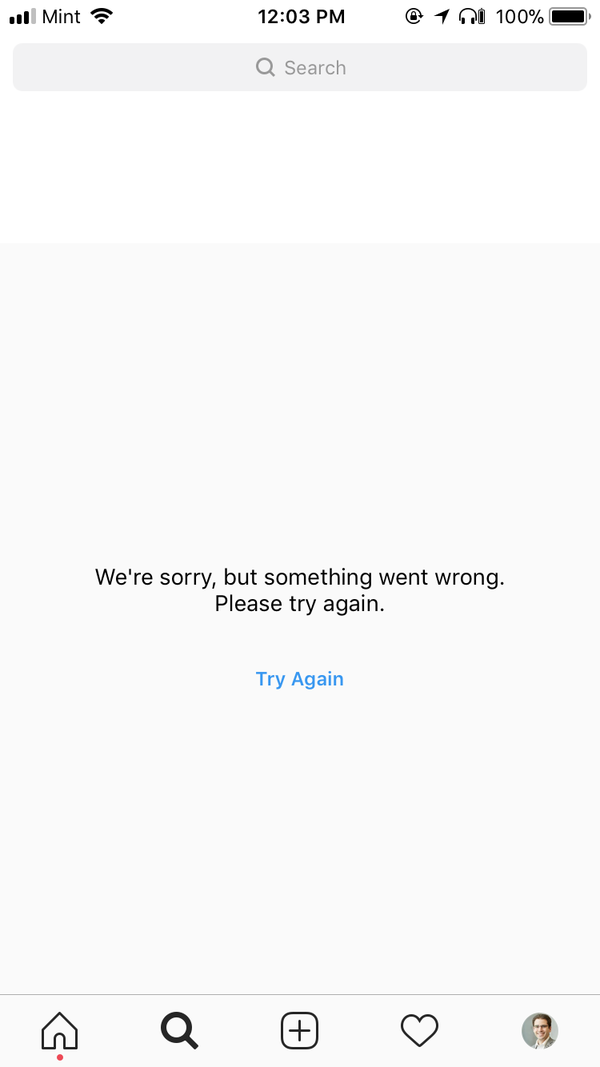The image is a vertical screenshot of a smartphone display, approximately two to two and a half times taller than it is wide. At the top left corner, there is a signal strength indicator showing three-quarters full, followed by the text "mint." To the right of the carrier information, the cellular data icon is displayed as fully active. Centered at the top, the time reads "12:03 PM." On the top right, there are several icons, including a 100% full battery indicator.

The background below the status bar is gray, with darker gray text and a magnifying glass icon labeled "Search" centered horizontally. Beneath this, on a light gray background and centered both horizontally and vertically, the message "We're sorry, something went wrong. Please try again." is displayed in black text. Below this message, in light blue text, the phrase "Try again" is also centered on the screen.

At the very bottom of the display, there is a horizontal line separating the main content area from the action buttons. The buttons, arranged from left to right, include a home icon, a magnifying glass, a square, and a profile icon. The profile icon resembles a professional image of a young man.